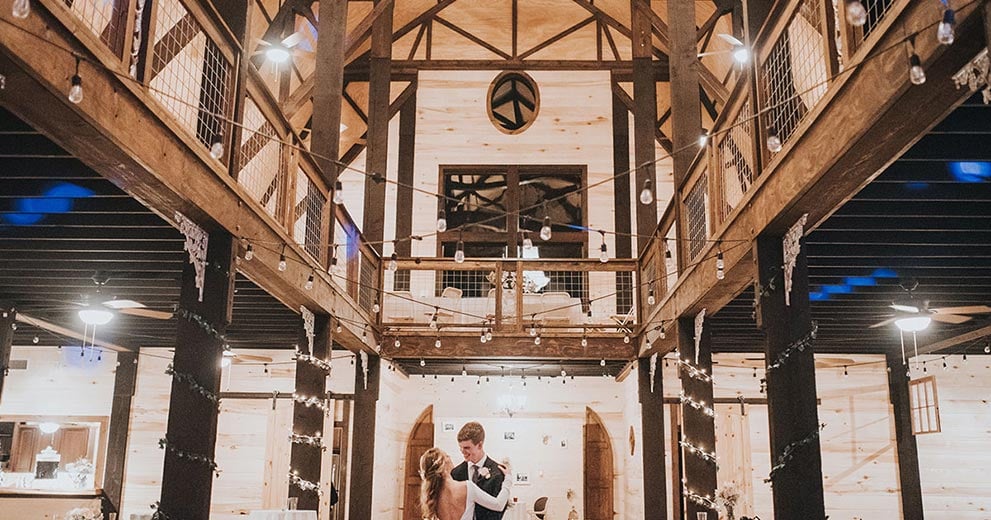The photograph depicts the interior of a multi-level wooden structure, resembling a large barn or rustic reception hall. The interior showcases exposed dark to light brown wood beams and framing, including substantial support beams on the ground level and an upper fenced layer. The wooden rafters stretch across the ceiling, contributing to the busy, open construction that reveals the intricacies of the structure. The space is festively decorated with white string lights wrapped around the wooden pillars and draped across the ceiling, casting a warm, incandescent glow.

In the center of the image, partially cropped, stands a bride and groom dancing. Facing away from the camera, the bride has long blonde hair cascading over her back and is wearing a sleeveless white gown that exposes her back down to the mid-section where the image cuts off. She has her arms around the groom, who has short brown hair and is attired in a black and white tuxedo adorned with a floral boutonniere on his left breast pocket. They are situated in front of two open barn doors, creating a picturesque and romantic scene.